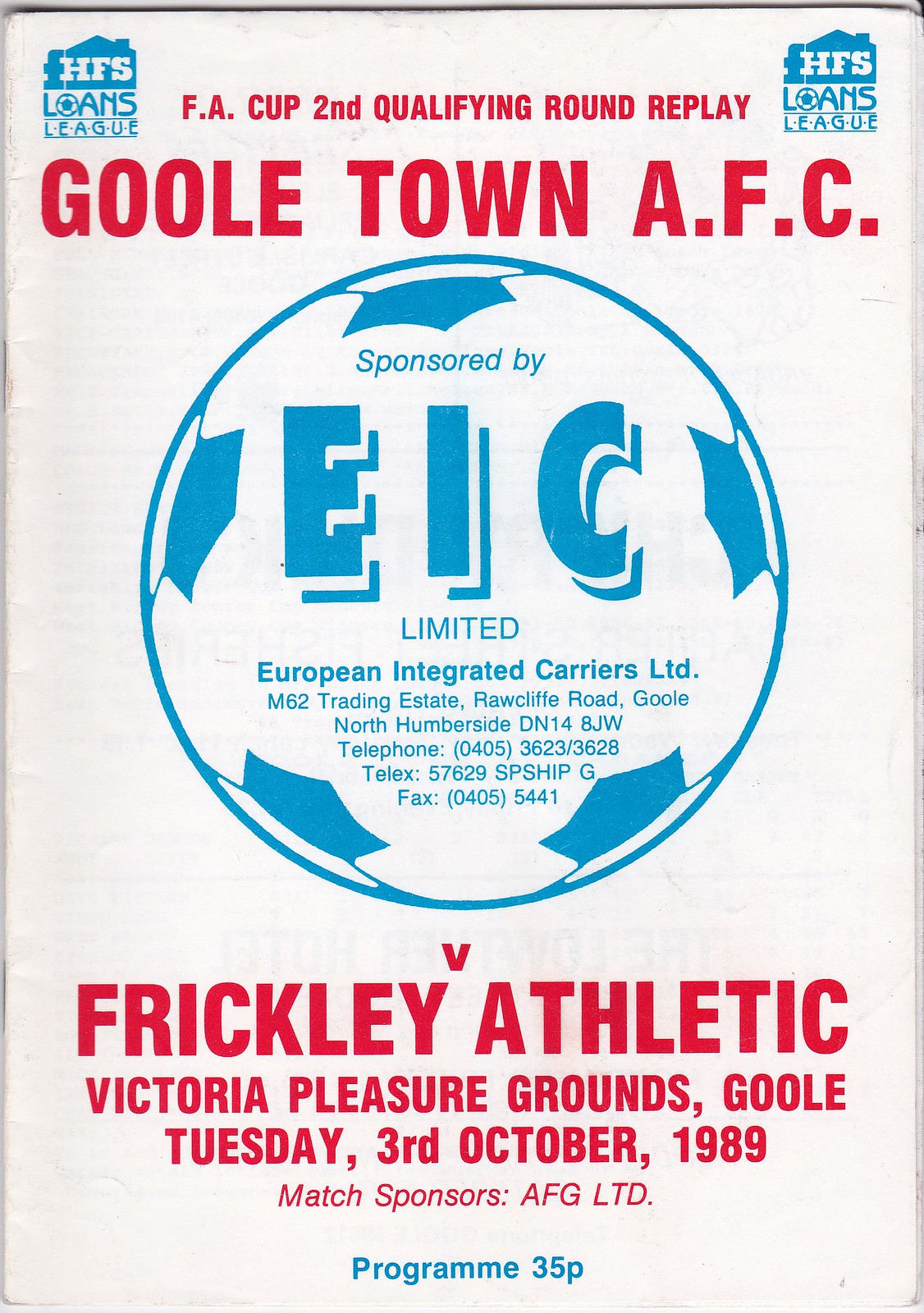The image showcases a detailed poster for a soccer event. The background is white, featuring the name "HFSS" inside heart-shaped logos on the top left and right corners. Centrally, it reads "F.A. Cup Second Qualifying Round Replay," with "Lone's Lodge" written below, where the letter 'O' is styled like a soccer ball. Further down, the poster highlights "GouldTown A.F.C." in prominent text. Below this, a blue-outlined soccer ball logo incorporates a pattern and the text "Sponsored by EIC Ltd." within it, extending to "European Integrated Carriers Ltd." and its address details: "M62 Trading Estate, Ratcliffe Road, Gould, North Humberside, DN14 8JW." A telephone contact is provided: "(0405) 3623 / 3628." At the bottom of the poster, "Frickley Athletic" is mentioned, indicating a match against GouldTown A.F.C. at "Victoria Pleasure Grounds," set for Tuesday, October 3, 1989. The sponsors include details about not just the match, but also "AFGLTD" programs.